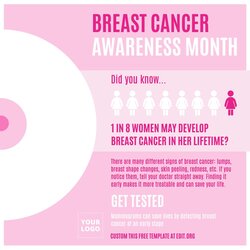This Instagram-ready infographic, shaped as a square, is designed to promote Breast Cancer Awareness Month. Set against a pink background, the focal point rests on the left side with three concentric circles: a small dark pink dot in the middle, encircled by a lighter pink ring, and finally, a white outer ring. At the top, bold text states "Breast Cancer Awareness Month."

Below, a lighter pink banner with the phrase "Did you know..." in darker pink text captures your attention. Underneath this banner, eight stick figure representations of women are displayed in a row. Seven of these figures are colored white, while the eighth figure stands out in pink, visually reinforcing the statistic presented below: "1 in 8 women may develop breast cancer in her lifetime." 

To further engage and inform, four additional lines of pink text follow this statistic, sharing vital information. At the bottom of the infographic, the imperative phrase "Get tested" is prominently featured in white text, encouraging proactive health measures.